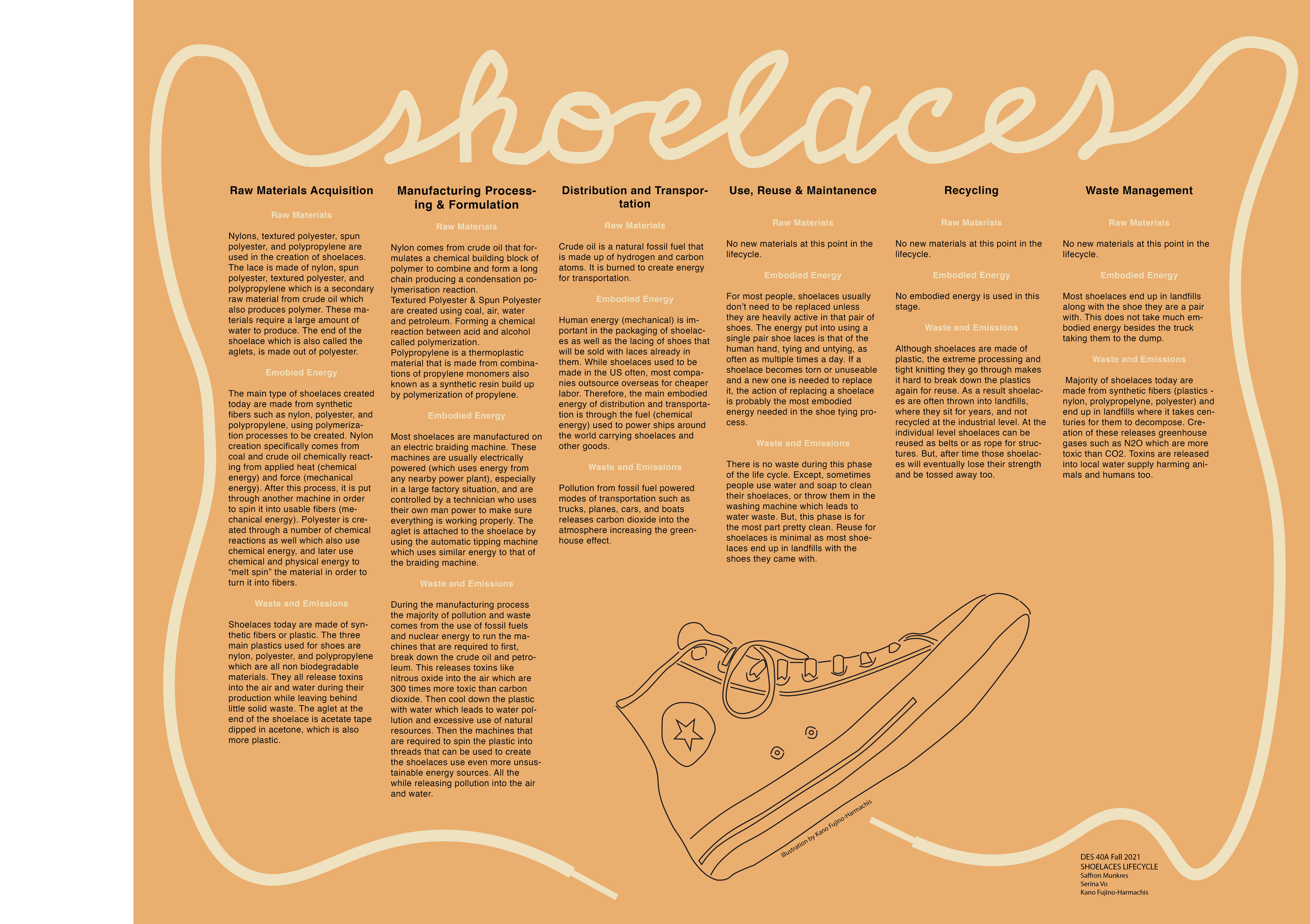The image features an informational poster with an orange background and the title "Shoelaces" written in cursive ivory-colored text. Gracefully flowing VS-like strokes extend from the 'S' at both ends, creating an elegant frame that encircles the entire image, mimicking the appearance of actual shoelaces. At the bottom, a minimalist black outline of a pair of sneakers adds a visual touch. The layout is organized into six distinct columns of text, each dedicated to a different aspect of the lifecycle of shoelaces. These columns include: Raw Material Acquisition, Manufacturing Processing, Distribution and Transportation, Uses Reuses and Maintenance, and Recycling and Waste Management. Each column is further divided into detailed sections with paragraphs that delve into topics such as embodied energy, waste, and emissions in the context of raw materials. This poster embodies a comprehensive overview of the production, usability, and environmental impact of shoelaces.